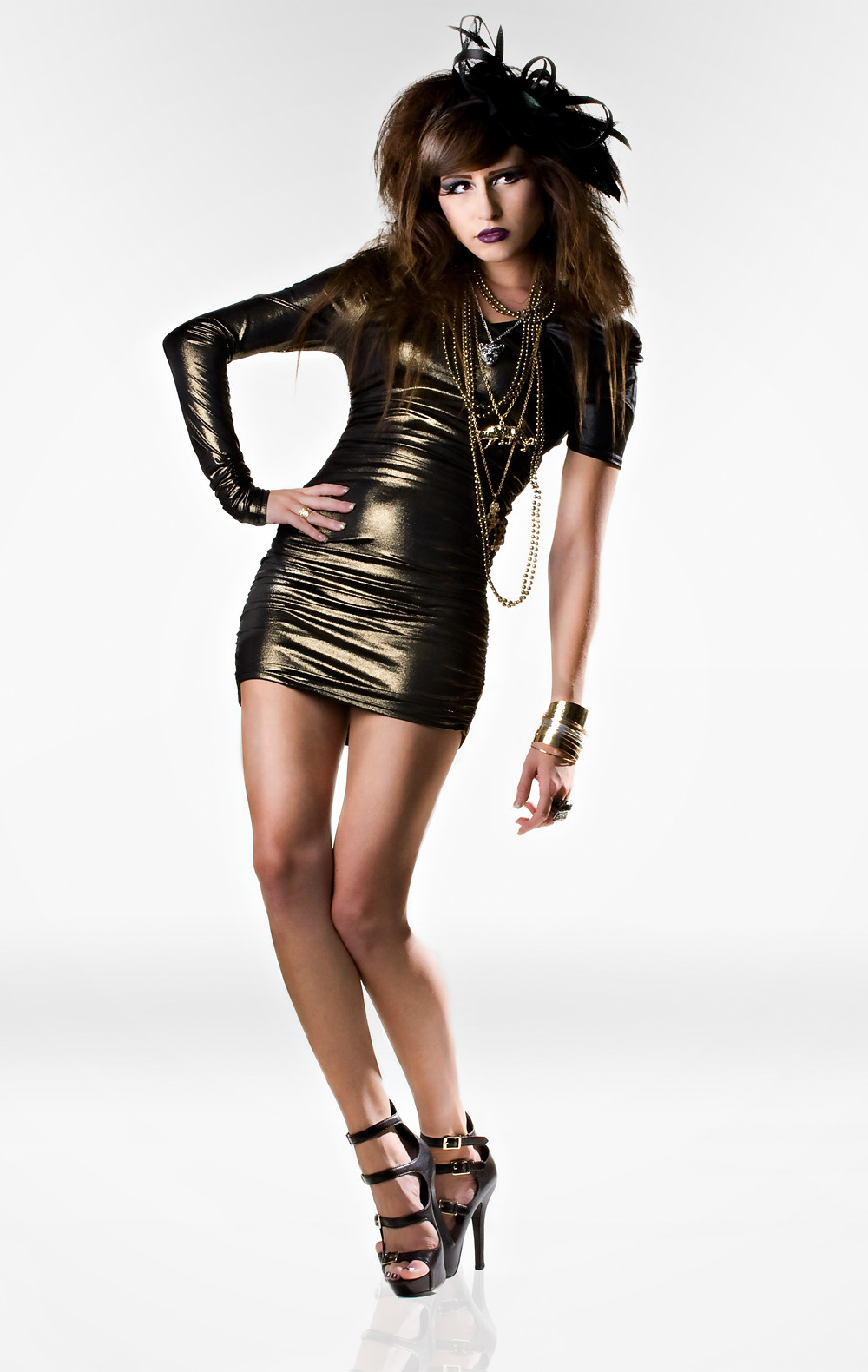The image showcases a striking photo of a woman posing against a completely white, photoshopped background where her faint reflection is visible at the bottom. She is dressed in a short gold dress, which is unique in design with asymmetrical sleeves: the right sleeve is long, extending slightly over her hand, while the left sleeve is cut above the elbow, rolling up to her shoulder. The dress appears very thin and silky smooth, with a light bluish-greenish tint, highlighting its delicate texture.

The model exudes elegance with her numerous accessories, including several golden rings and bracelets on her left wrist. Around her neck, she wears an abundant collection of necklaces, at least a dozen, featuring various designs and lengths, with some necklaces adorned with gold animals and one being silver.

Her footwear consists of black high-heeled open-toed shoes, styled with multiple sandal-like straps—four of them—leaving much of her foot visible. 

Her brown, voluminous hair is styled with a frilly black, feathery headdress, adding a dramatic touch. She complements her look with bold makeup: dark purple lipstick and winged eyeliner that accentuates her eyes. Striking a confident pose, she places one hand on her hip, making for a compelling and fashionable image.